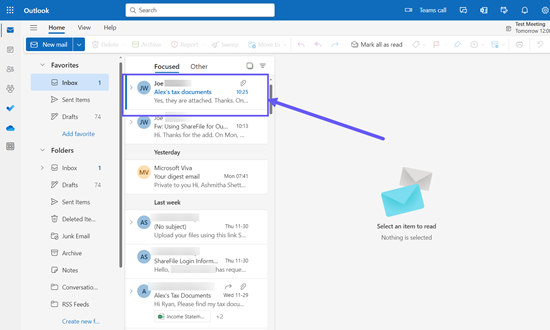The image depicts a horizontal rectangular Outlook email interface with a blue header bar running from left to right along the top edge. In the upper left corner of this blue bar, there is a white Outlook logo and near it, slightly to the left, resides an icon. Centrally positioned within the blue bar is a white search box, flanked by additional icons on the upper right side.

Below this header, the background transitions to light gray. Along the left column, various icons are displayed, leading into a horizontal menu featuring tabs labeled "Home," "View," and "Help." Adjacent to this, another blue horizontal area contains a drop-down menu labeled "New Mail" in white text.

Under the blue area, sections titled "Favorites" and "Folders" are displayed in bold black font. The "Favorites" section includes sub-items such as Inbox, Sent Items, Drafts, and a turquoise "Add Favorite" option. The "Folders" section similarly lists Inbox, Drafts, Sent Items, Deleted, Junk Email, Active, Notes, Conversation, RSS Feeds, and a turquoise "Create New" option, each accompanied by respective icons to their left.

At the top of the main content area, two tabs labeled "Focused" and "Other" in black bold text underlined in purple separate different sections of emails. Below this, individual email items appear, each prefixed by a colored circle containing initials, followed by the sender's name in black and a brief email description in turquoise. The first email item displays a circle with "JW," the name "Joe," and the subject "Alex's tax documents," followed by "yes, they are attached thanks."

Highlighted by a purple rectangle, with an arrow extending from the gray background pointing towards this specific email, the focus is drawn to this area. Lower down on the right-hand side, there are icons depicting envelopes, with the prompt "select an item to read" displayed adjacent to them. The overall design emphasizes an organized, user-friendly layout typical of an email client interface.